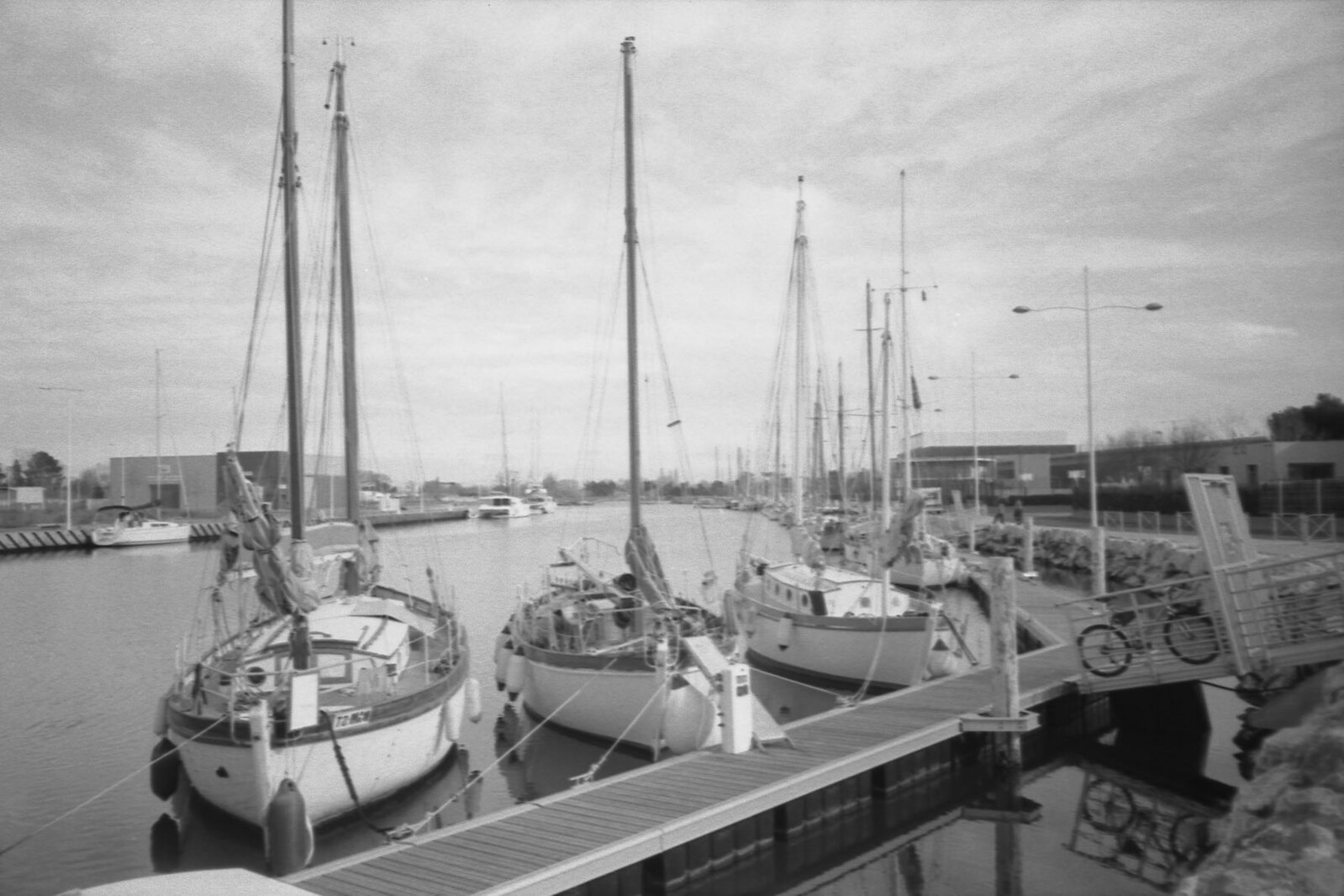This black-and-white photograph captures a tranquil waterfront scene. At the center of the image, three sailboats are moored at a narrow, timber wooden dock, positioned diagonally from the bottom left to the middle right. The boats are facing the viewer head-on, with their tall masts standing proudly but their sails neatly tucked away. The boat on the left features two masts, while the one in the center has a single mast. 

In the background, a broad waterway stretches into the distance, appearing to be a river. On the far side of the river, buildings and clusters of trees are visible, creating a scenic contrast between nature and architecture. The left side of the riverbank also hosts some structures, while on the right, power lights and a square building can be seen beyond a rocky bank and a road. 

A tiny boat is spotted towards the middle of the water, with an additional boat faintly visible on the left. In the bottom right corner, there's what seems to be a steel crate containing two round objects, and nearby, a bicycle is approaching the scene. The sky overhead is filled with stratified clouds, casting a gray, serene mood over the entire landscape.